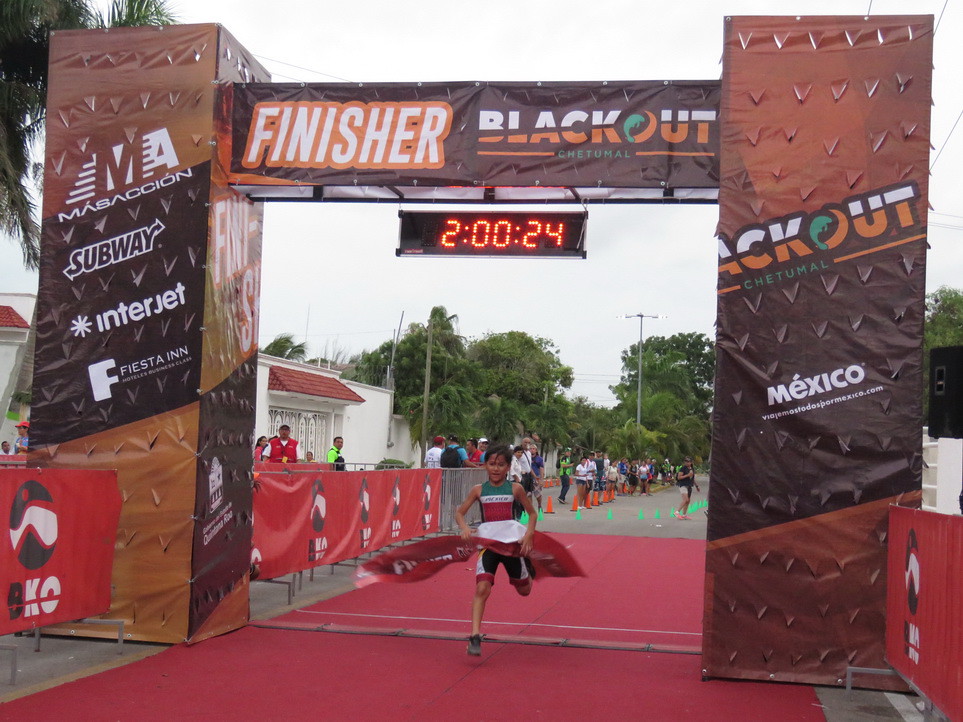In this vibrant outdoor scene captured in the middle of the day, a runner is seen triumphantly approaching the grandiose finish line of a race in Chetumal, Mexico. The event is marked by two imposing rectangular pillars, decorated in earthy tones of brown and black, and adorned with a distinctive spiky design of partially peeled plastic triangles. These pillars frame an archway overhead that proudly displays the text "Finisher" and "Blackout, Chetumal, Mexico" in bold white letters with an orange border. Below the arch, a digital timer reads "2:00:24," indicating the runner's finishing time. The ground beneath is a typical asphalt road, with a striking red carpet extending towards the finish line, adding a touch of elegance and festivity. Numerous sponsors, including Subway, Massasyon, Interjet, and Fiesta Inn, are visible on the left side of the image. In the background, walls and cones fence off the crowd, maintaining order as the runner, dressed in athletic gear, makes his way directly under the arch, positioned centrally in the image. The colors in the image span from gray, maroon, and red to black, white, lime green, orange, brown, blue, and green, creating a vivid and dynamic representation of this exciting moment in the race.